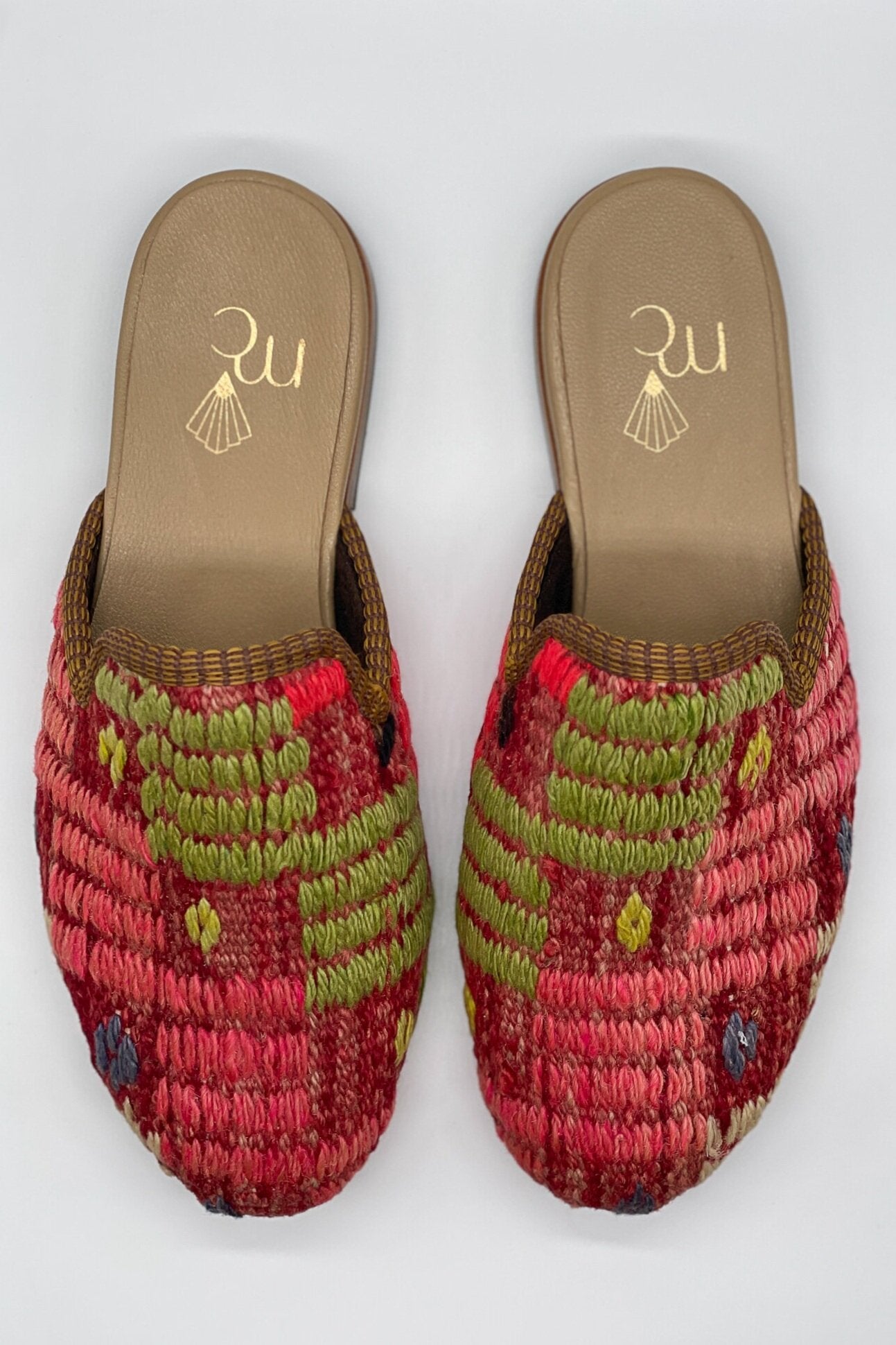This bird's-eye-view photograph showcases a pair of closed-toe, slip-on sandals laid side by side, with the front of the shoes oriented towards the bottom of the image and the back towards the top. The background is a flush gray color which contrasts with the intricate design of the sandals. The soles of the shoes are light brown, resembling leather, and feature a gold inscription that reads "MC," accompanied by a fan-shaped logo. The upper part of the sandals is crafted from a textured material that appears to be yarn or tweed. This material is arranged in a patchwork of various colors, predominantly dark green, dark pink, crimson red, dark red, and fuchsia, interspersed with splotches of yellow and blue flowers, creating a visually engaging and eclectic design.